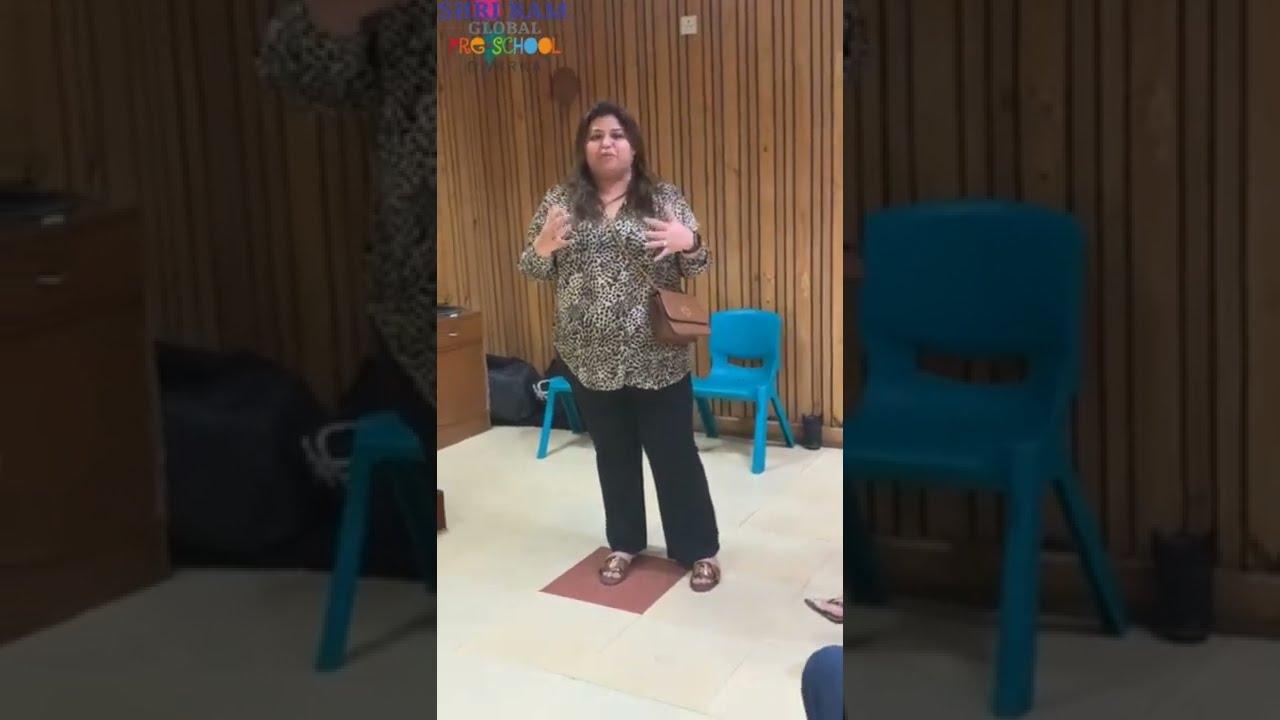In the image, a woman with lighter brown skin and fluffy, straight brown hair that falls just past her shoulders stands facing the camera on a white floor, precisely inside a reddish rectangle. She is wearing a black and white leopard print blouse paired with black slacks and brown open-toed sandals. Draped over her left shoulder is a brown purse. The woman, who appears to be of Hispanic or Mexican descent, has a full, plus-sized figure and a friendly demeanor, suggested by her slightly expressive hands held in front of her chest as if she is speaking.

Behind her, two blue child-sized chairs are arranged in front of a brown wooden wall. To the left side of the image, there's a small cabinet with a red and navy blue bag behind it and a sign above that reads “global preschool” in white and multicolored text. This sign is partially obscured by the background color. The image is framed by two blurred, darkened segments on the left and right, which are actually enlarged, blackened sections of the same picture. On the right, there's a discernible part of someone’s leg and foot, while the left side shows an up-close view of the background behind her. This structured composition hints at a classroom setting and adds depth to the scene.